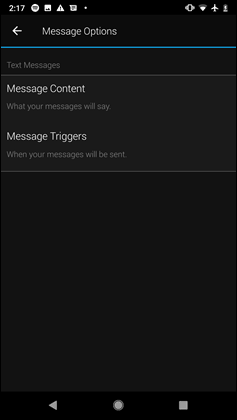The image showcases a smartphone screen with a user interface for configuring automated message settings. The background is black, and all text is written in white. At the top of the screen, "Message Options" is displayed next to a white back button on the left. Directly beneath this header is a thin line that transitions from blue to pink and back to blue.

Below this line, the text "Text Messages" introduces the main sections. The first section, labeled "Message Content," describes where users can enter or select the message that will be sent automatically. The subsequent section, "Message Triggers," explains the conditions under which the message will be sent. This means the designated message will only be sent when a predefined event or condition (trigger) occurs.

This detailed layout of the screen ensures that users understand they can automate their messaging based on specific triggers, and the message content they define will be delivered accordingly.